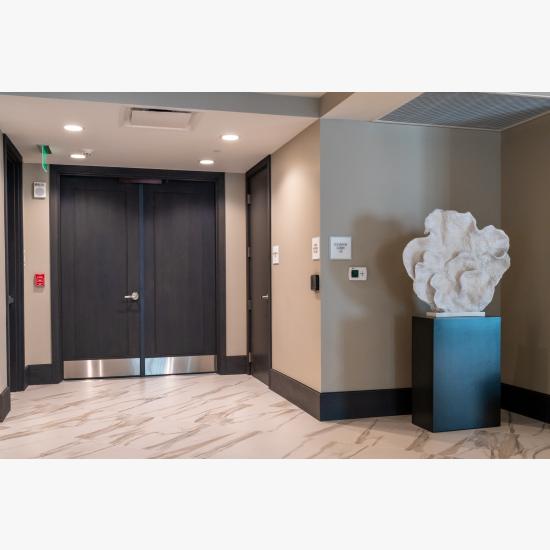The image depicts a modern indoor hallway, potentially located in an office, apartment, or business building. Central to the scene is a set of black double doors at the end of the hallway, identifiable by silver rectangular accents at the bottom and a silver handle. To the left of these doors, a red fire alarm pull is visible along with a green exit sign hanging from the ceiling. Above, bright white halogen lights illuminate the space, casting a warm glow despite the otherwise sterile surroundings. The floor features light beige, almost marble-like tiles with intermittent brown markings. The walls are beige with black moldings at the floor's base, adding contrast. On the right side, near a corner, stands a black pedestal supporting a wavy white sculpture reminiscent of coral. There is also a mention of another doorway on the left wall, partially hidden from view. Overall, the clean lines, contrasting colors, and detailed elements of the stairwell sign, lighting, and sculpture contribute to the sleek, formal aesthetic of the hallway.